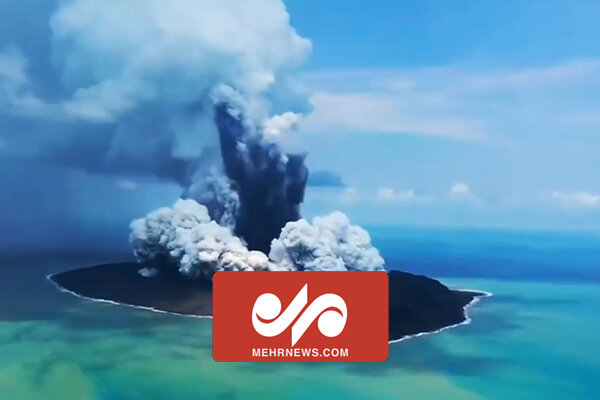The image depicts a dramatic volcanic eruption on a small, remote island in the middle of an aqua-blue ocean. The scene is dominated by a massive explosion at the island's center, with thick black smoke billowing upwards. This central plume of black smoke is surrounded by expansive clouds of white smoke, forming a large, chaotic mass, blending into the blue and white sky in the background. The entire image has a surreal, almost creamy and soft-filtered appearance. Situated in the foreground of the image, there's a red rectangle with smooth edges, displaying the text "MEHRNEWS.com" in white, prominently standing out against the scene's natural chaos.